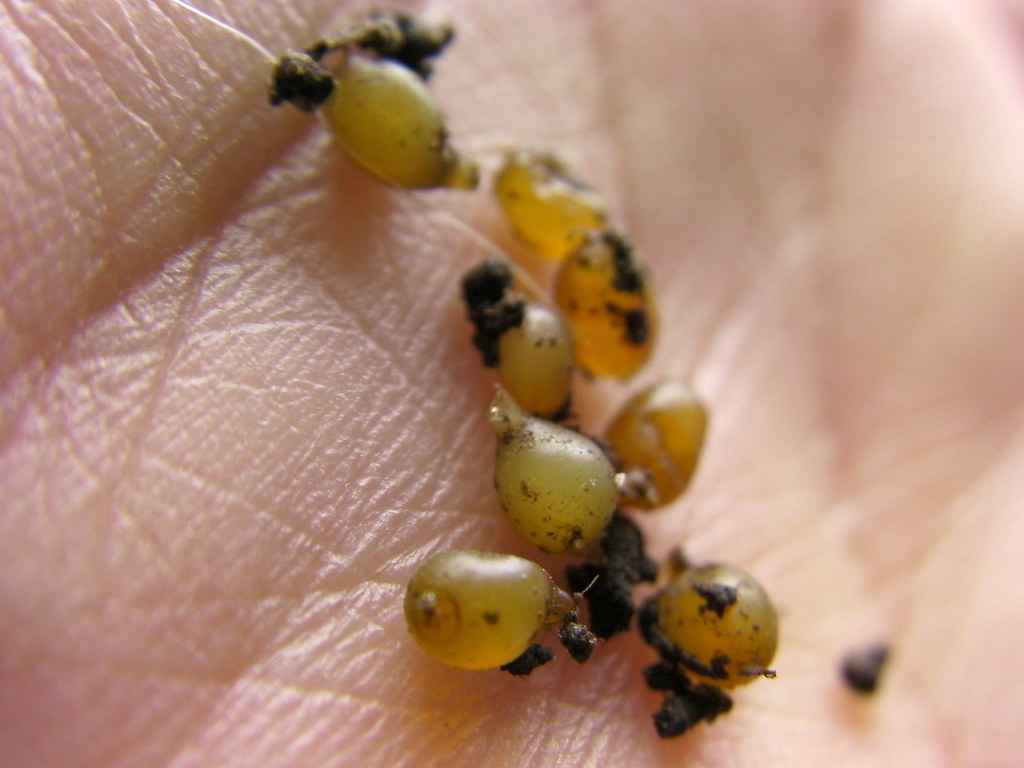The image is a large, square close-up photograph of the palm of a person's hand. The hand is predominantly beige and features detailed, visible lines, especially on the left side where it's in focus. The right side of the hand is blurry, but the palm's lines are still discernible. In the center of the image, from top to bottom, there are several small, round, light green objects that resemble grapes, numbering around eight. These grape-like objects appear shriveled and covered with small brown fragments, resembling dirt crumbs. Each object has a distinctive head-like protrusion, which could be mistaken for stems or perhaps nozzles, making them appear as if they were freshly pulled from the soil.